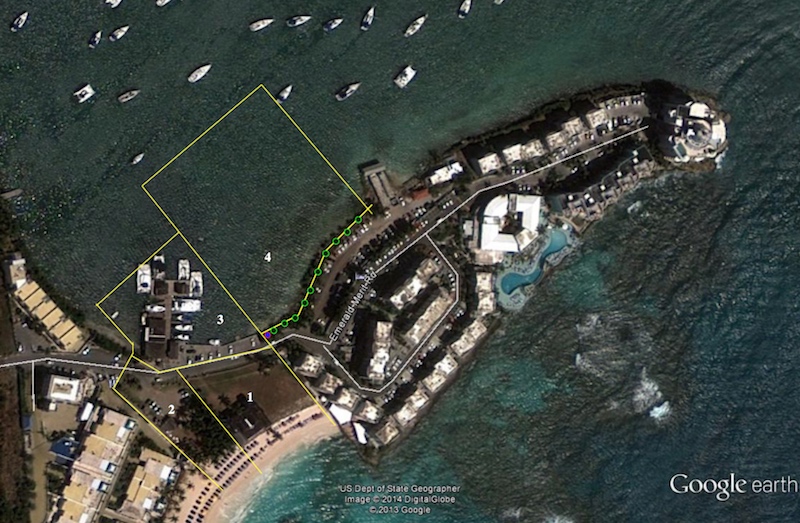This vibrant and detailed overhead satellite image, taken from Google Earth, captures a coastal town prominently situated on a thin peninsula that juts into the ocean. The photorealistic depiction shows the peninsula extending from the bottom left to the top right of the frame, resembling a finger extending from a hand. The landscape is densely packed with suburban buildings, including a distinct square building in the center, tilted like a diamond, and a large structure at the peninsula's tip. Numerous shiny, white-topped motorboats and sailboats can be seen moored in the bay at the top left corner of the image, creating a mosaic of maritime activity. 

Notable in the scene are several yellow grid squares, possibly indicating developmental plans or areas of interest. One larger, jagged-edged grid sits on the left side of the landmass, with smaller squares nearby, denoting docks with boats. On the bottom left corner, the peninsula connects to a larger landmass featuring visible buildings and a sandy beach to the right. 

The deep blue shades of the open ocean envelop the scene on the bottom right, contrasting with the vivid green dots indicating ongoing construction plans within the largest yellow grid. In the lower part of the image, small white text reads "U.S. Department of State Geographer Image © 2014 Digital Globe © 2013 Google" and "Google Earth," marking the authenticity and origin of the satellite view. The image is a testament to the seamless integration of natural and developed landscapes, providing a comprehensive visual of the bustling coastal town.